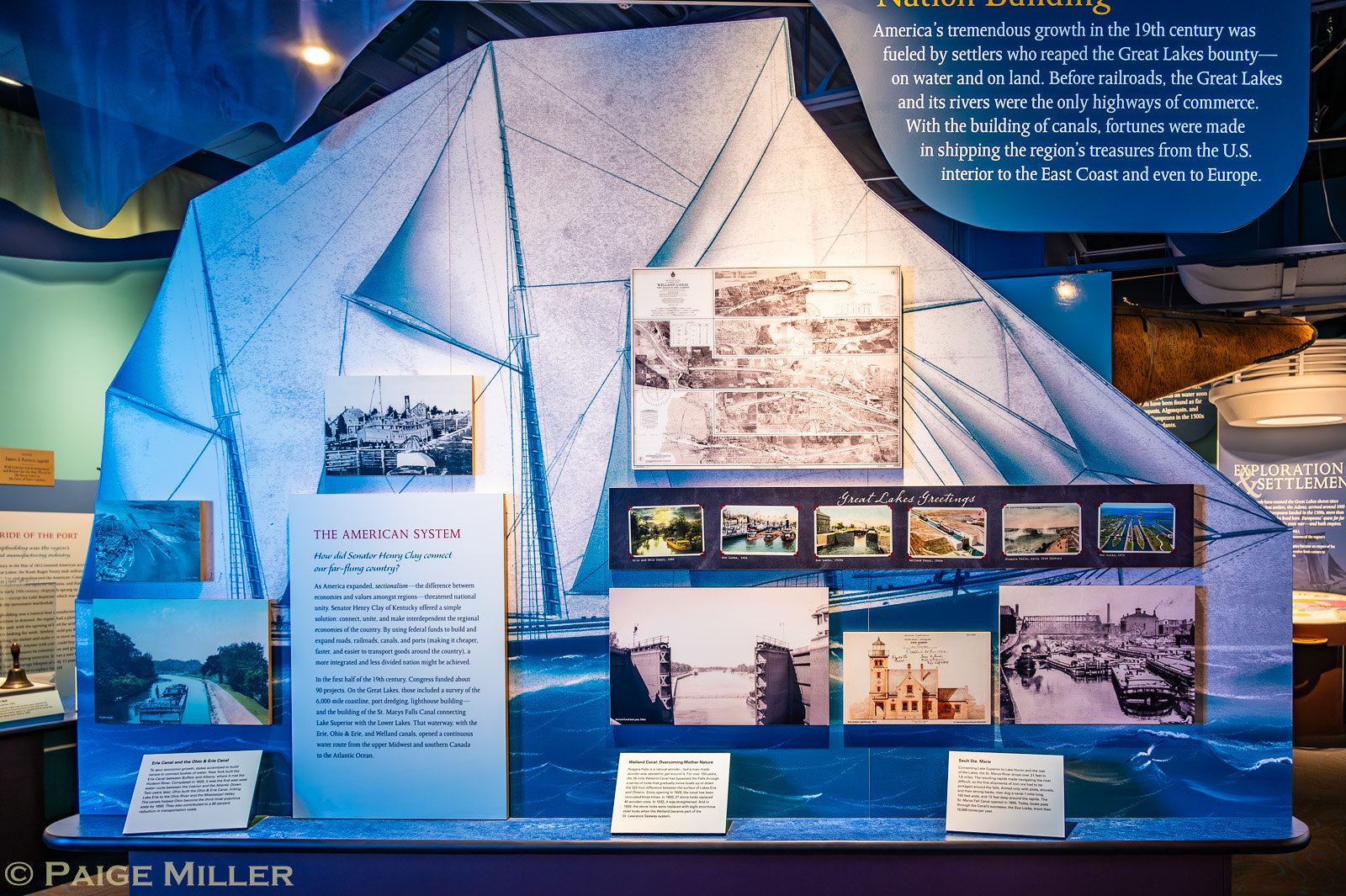The image is a detailed display, possibly an advertisement or exhibit, highlighting the Industrial Revolution in the United States during the 19th century. This horizontal rectangular display features a prominent white coat or jacket centered with no person wearing it. To the right, there are various photographs—large ones at the bottom and smaller ones along the top—accompanied by explanatory text. The upper right corner of the display contains a blue background area with a lot of white text, some of which reads, "America's tremendous growth in the 19th century was fueled by settlers who reaped the Great Lakes' bounty on water and on land. Before railroads, the Great Lakes and its rivers were the only highways of commerce. With the building of canals, fortunes were made in shipping the region's treasures from the U.S. interior to the East Coast and even to Europe."

The backdrop of the display includes the distinctive image of a large sailing ship with its sails extended. There is a notable vertical placard, about three to four feet tall, declaring "The American System" in red letters. Further down, a placard with text and a photograph offers additional details about the exhibit. The right bottom section of the display features a sign stating "Exploration Settlement" in white letters on a blue background. The background scenery includes what appears to be a wall and possible flight of stairs. The name of the photographer, Paige Miller, is visible in the lower left corner against a brown and blue background.

In essence, the display serves as an educational piece on America's Industrial Revolution, emphasizing the transformative role of waterways and canals in the 19th-century economic boom.